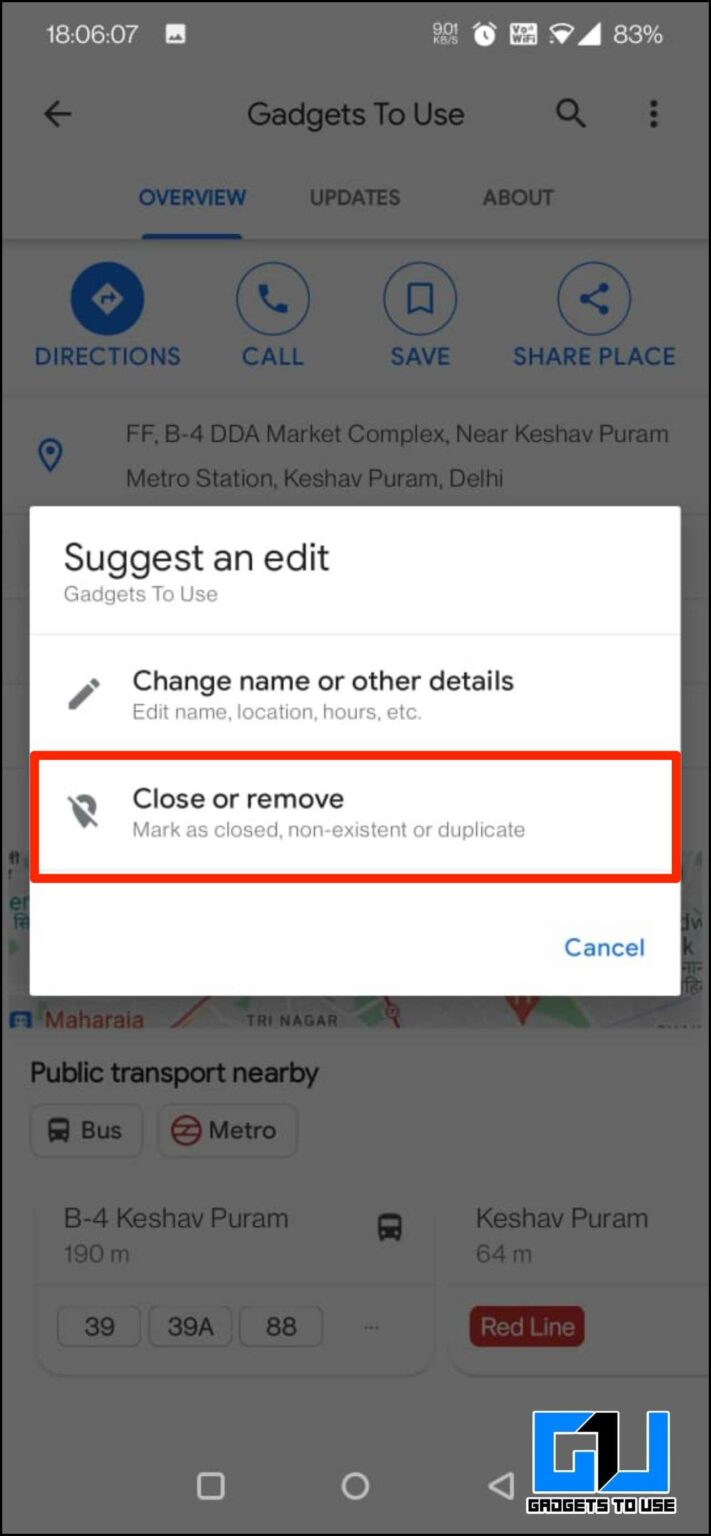The image displays a screenshot taken from a mobile device, specifically while using the Google Maps app. The background features a grayed-out image with various elements, but the focal point is a pop-up box centrally positioned in the foreground.

The pop-up box is titled "Suggest and edit gadgets to use." Below the title, there is a pencil icon indicating editing capabilities, accompanied by text that reads, "Change name or other details, edit name, location, hours, et cetera." Directly beneath this, another option displays a map pin symbol with a strikethrough, labeled "Close or remove," and explains, "Mark as closed, nonexistent, or duplicate." This section is highlighted in red. In the bottom-right corner of the pop-up, a "Cancel" button is visible.

In the background, the top of the screen shows it is a Google Maps selection, displaying the title "Gadgets to use." To the left of this title is a back arrow, and to the right is a magnifying glass icon. Below these navigation icons, there are three tabs labeled "Overview," "Updates," and "About," with the "Overview" tab currently selected.

Further down, a set of action buttons are visible, offering options for "Directions," "Call," "Save," and "Share." Below these buttons, the text indicates the location as "FFB4DDA market complex, near Kashavpuram metro station, Kashavpuram, Delhi." The map itself is shown underneath this description but is mostly obscured by the pop-up box. Finally, there is a note about public transportation options nearby: "Bus or metro, B4, Kashavpuram bus station, 190 meters."

At the very bottom of the screen, the typical phone navigation buttons for "Menu," "Back," and "Home/Selection" are displayed.